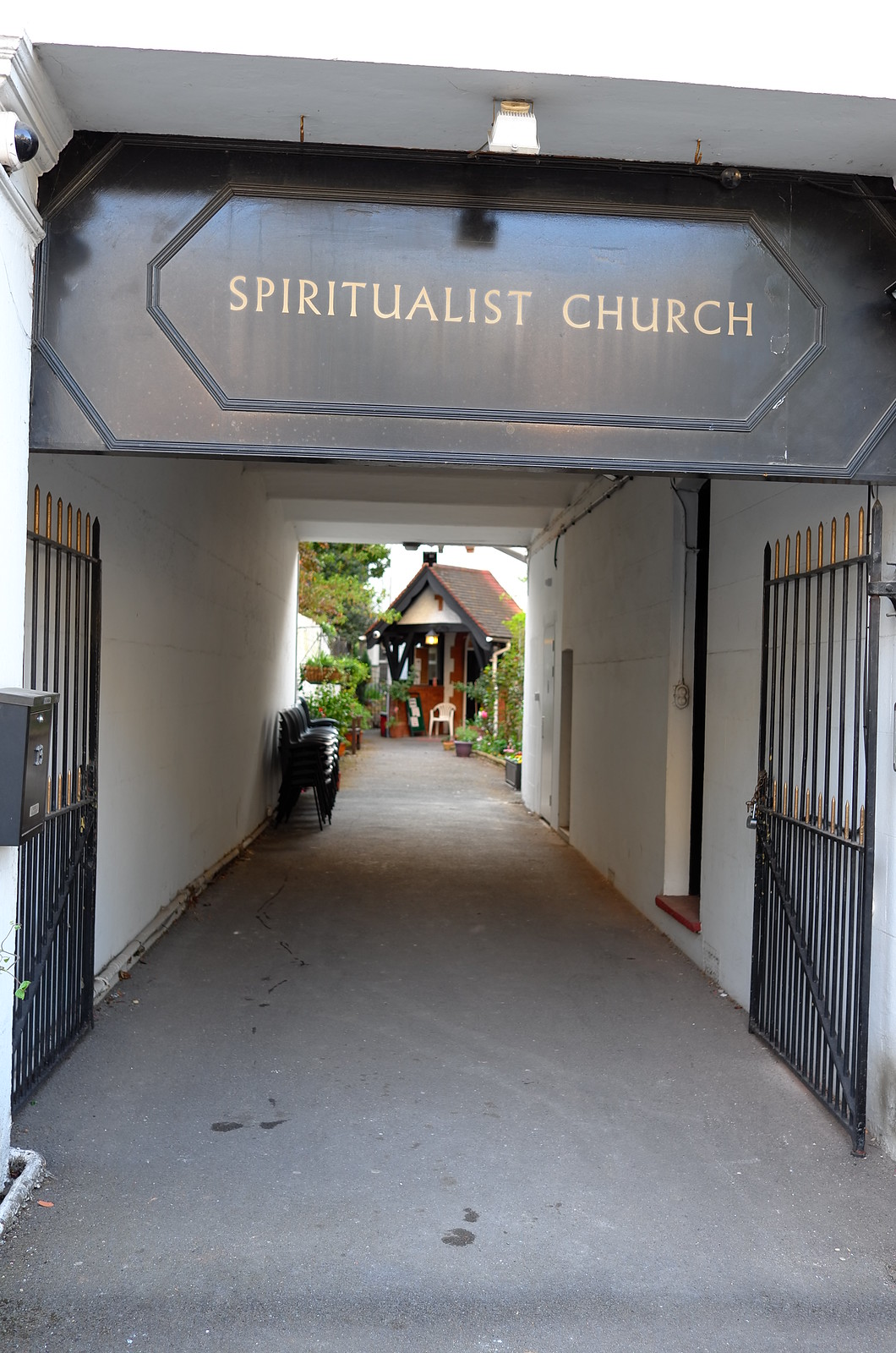The image showcases the entrance to the Spiritualist Church, with the sign "Spiritualist Church" prominently displayed in gold letters against a dark black background. The entrance pathway is flanked by black metal gates that open up to an alleyway or breezeway, leading towards the back of the premises. This pathway has a typical grey floor with a couple of darker markings.

The alleyway, which is enclosed by a white-walled corridor, guides the viewer's eye to a door in the background. This door seems to be connected to a smaller building, potentially a worship or meditation center, and is accompanied by a brown rooftop visible from this vantage. Green bushes and trees frame the background, adding a touch of nature to the scene.

To the left side of the corridor, there appears to be a stack of chairs and a black post box, marked with the number 13 in silver. Additionally, there's a black camera in the top left corner monitoring the entrance. Near the door, you can spot some seating arrangements and a white seat by the door under an awning with the number one on it. The combination of architectural elements and garden features creates a tranquil yet structured entrance to the church.